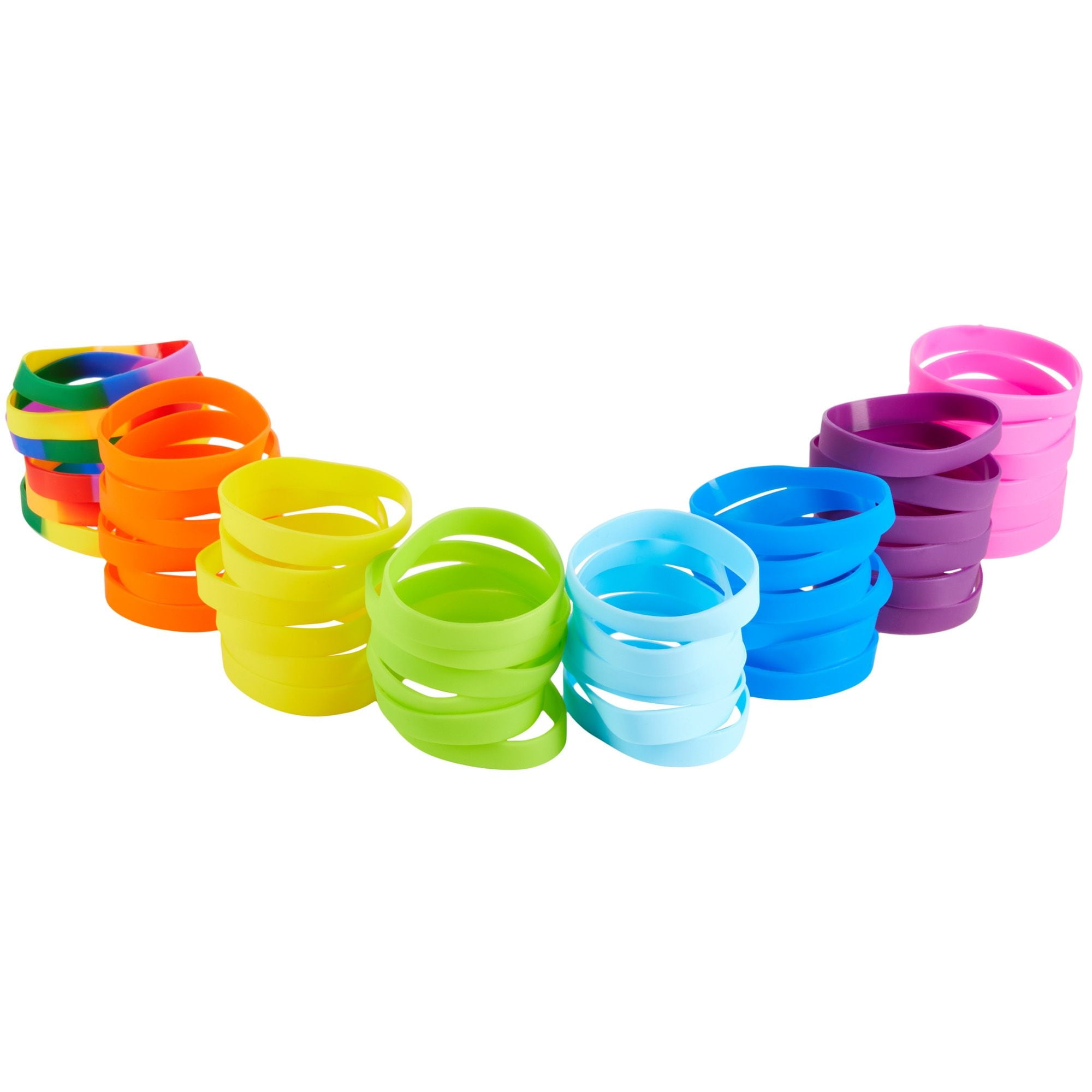This stock photo captures an assortment of colorful silicone bracelets, typically handed out at events or schools. The bracelets are loosely arranged in an L-shaped pattern, forming a corner of a square against a white backdrop. Starting from the top left, the first set of bracelets features a vibrant rainbow pattern including green, blue, pink, red, and yellow hues. Next to them, a batch of solid orange bracelets is visible. Following this are stacks of yellow, green, light blue, blue, purple, and pink bracelets. Each color set contains roughly five to six bracelets, stacked in a manner that creates a half semicircle shape. The colorful display highlights the playful and slightly disorganized arrangement of the silicone bands, showcasing their varied shades and tones.